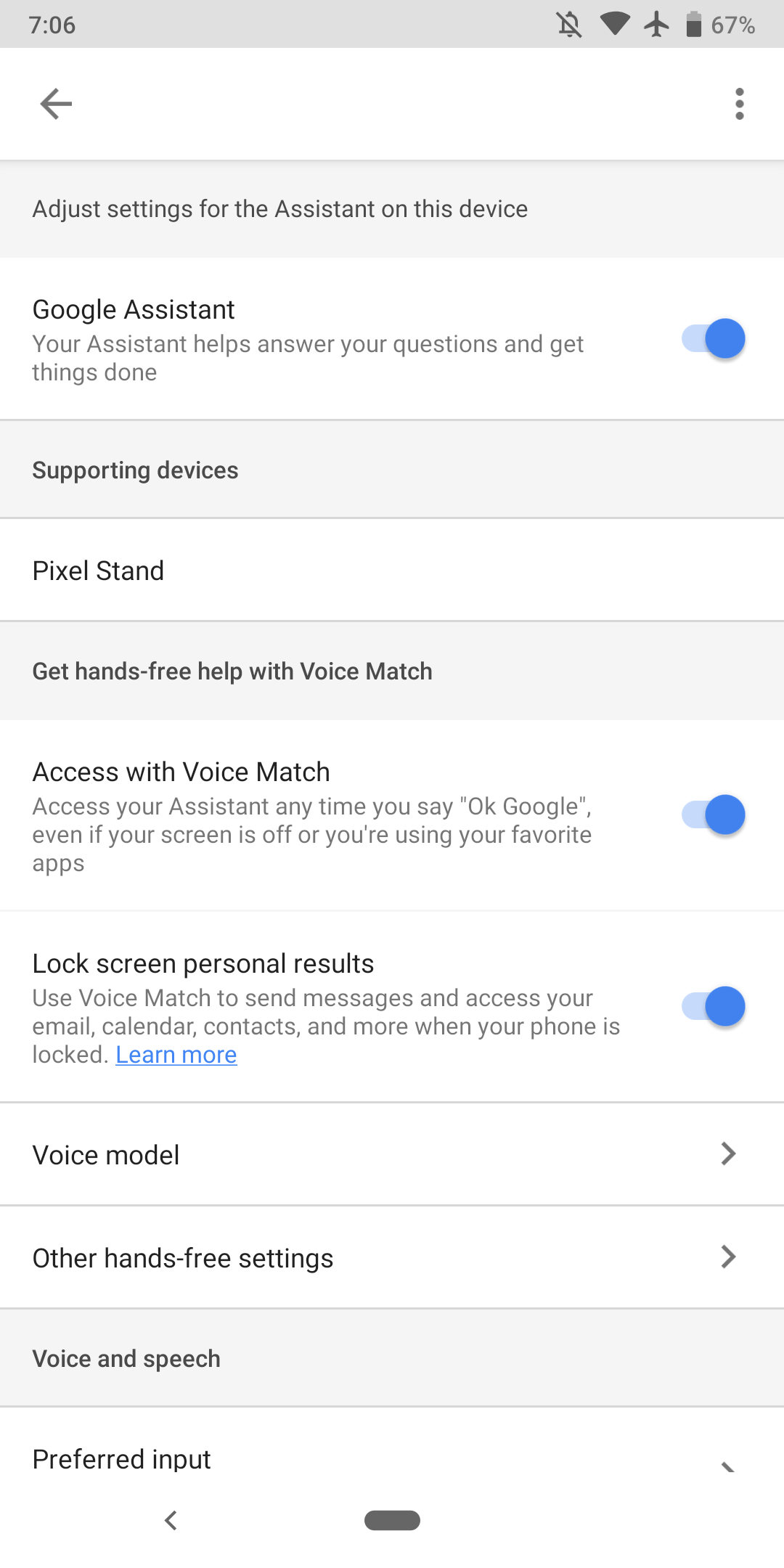This screenshot captures the settings page for Google Assistant on a mobile device. 

At the top, the status bar shows the current time as 7:06, a battery life of 67%, and indicators for airplane mode and a Wi-Fi connection. The alarm is turned off. 

Below the status bar, the screen features a navigation bar with a back arrow on the left and a three-dot menu on the right. 

Centered below this in a darker gray section is the text: "Adjust settings for the Assistant on this device."

Following this, on a white background, is the heading "Google Assistant," accompanied by the description: "Your Assistant helps answer your questions and get things done." To the right of this description is a toggle switch that is turned on, indicated by a blue circle.

The next section is titled "Supporting devices," with "Pixel Stand" listed underneath. Below this, you see "Get hands-free help with Voice Match," which includes options that can be toggled on or off.

The first option is "Access with Voice Match," which allows the Assistant to be activated by saying "Okay Google," even when the screen is off or apps are in use. This option is switched on.

The second option is "Lock screen personal results," which uses Voice Match to send messages and access email, calendar, contacts, and more while the phone is locked. A "Learn more" hyperlink is provided for additional information, and this option is also toggled on.

Further down, you see "Voice model" and "Other hands-free settings." The last section, "Voice and speech," displayed on a gray background, precedes the final item, "Preferred input," on a white background.